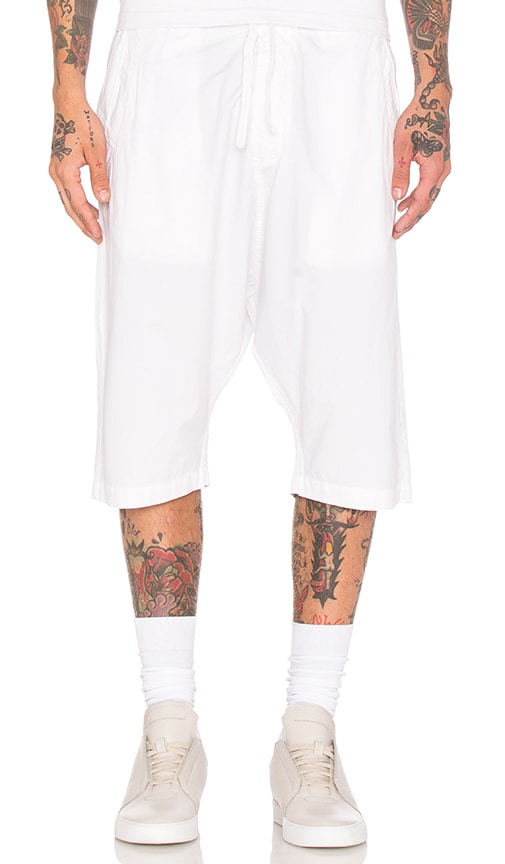The image captures the lower half of a light-skinned male model, showcasing his tattoos and outfit. He is attired in bright white, loose-fitting shorts that extend just past his knees, resembling capri pants, with a visible drawstring. His legs are partially exposed from the knees to mid-calf, revealing intricate tattoos. On his left leg, there's a large rose tattoo, while his right leg features a dragon with a figure climbing up it. His arms and hands also have detailed tattoos, including a skull, a flower, and various designs with colors such as greens, reds, purples, and blues. The model is also wearing clean, white tennis shoes, white socks, and off-white high-top sneakers which appear khaki-colored. The reflection of the shoes is seen at the bottom of the image.